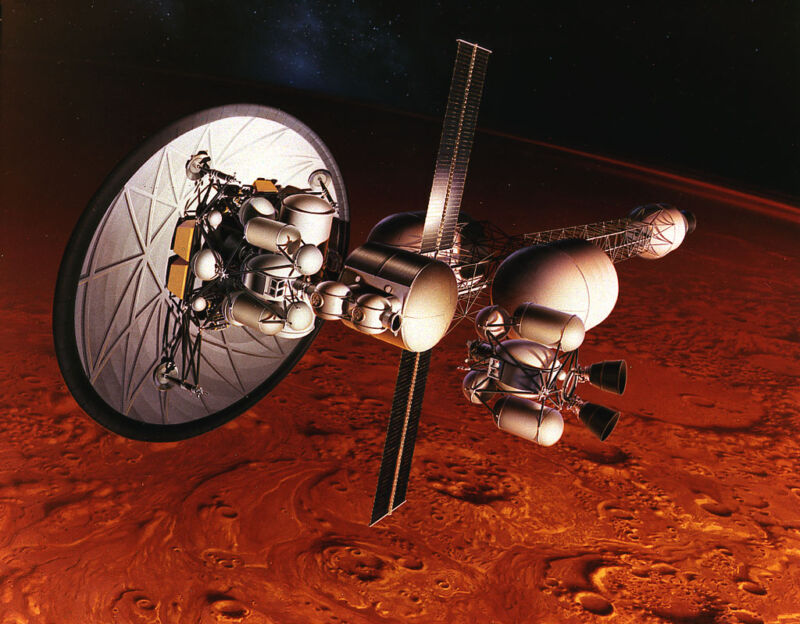The image is a detailed color photo, potentially an artist's rendition, of a sophisticated satellite orbiting Mars. The satellite features a large, circular silver disc on its left side, which prominently supports several components, including a dome-like structure with an attached thruster. Extending from the central body, rectangular solar panels stretch vertically above and below the satellite, enveloped by a metal lattice grid structure. A pill-shaped container is also noticeable, contributing to the satellite's intricate design. Mars, the red planet below, is depicted with a striking reddish-orange surface covered in numerous craters, suggesting heavy impact activity. The background unveils the vast dark expanse of space, dotted with white stars and accented by a bluish galaxy-like cloud in the upper left, enhancing the cosmic ambience of the scene.